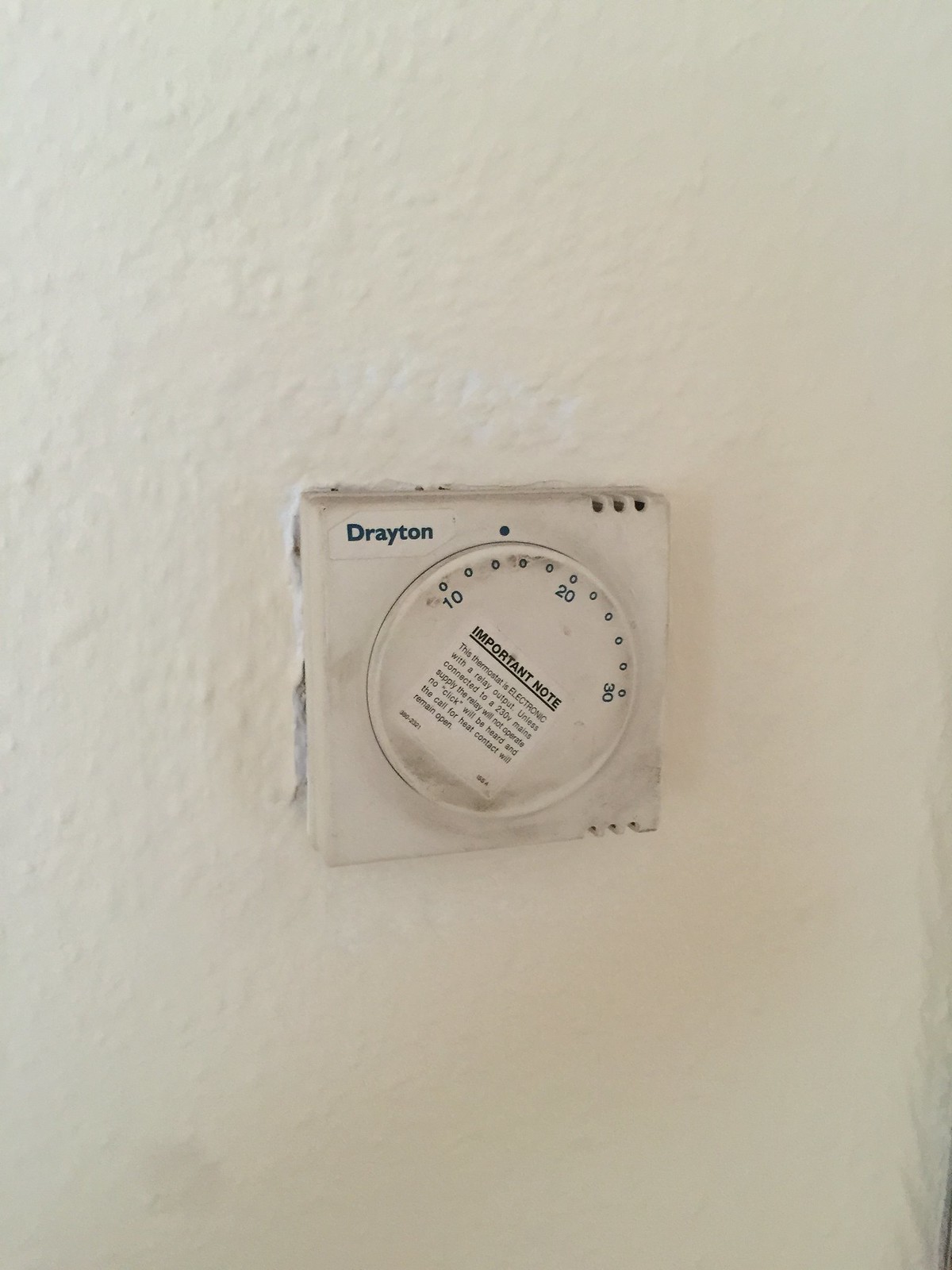The photograph captures an aged and slightly grimy electronic thermostat mounted on a beige wall. The thermostat is branded "Drayton," with the name clearly displayed in the top left corner of the device. It features a circular dial at its center, marked with numbers 10, 20, and 30, with the current setting appearing to be around 13. The device looks quite old, with noticeable dirt and brown discoloration, especially around the bottom of the dial.

A detailed instructional note on the thermostat indicates that it is electronic with a relay output, requiring a 230 V main supply to operate correctly. The message warns that without this connection, no clicking sound will be heard and the call for heat contact will remain open.

The wall behind the thermostat shows signs of wear and installation damage, with visible cracks on the left side and the right corner near the device. Additionally, there are three small black holes located in both the top right corner and the bottom of the thermostat, possibly indicating where it was previously mounted or additional adjustments made during installation.